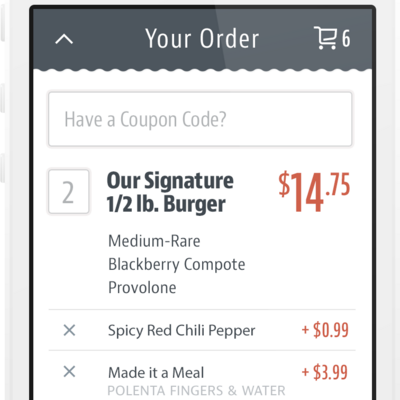**Detailed Caption:**

The image is a vertically oriented rectangle with a prominent gray border on the left and right sides, thicker than the thin gray border along the top. On the very left, vertical gray dashes are visible. Inside the top part of the image, encased within the gray border, is a thin black border that frames the top and sides of a horizontally placed gray banner. 

The gray banner features a white upward arrow on the left side. In the center of the banner, the text "Your Order" is prominently displayed, while on the right side, there is a shopping cart symbol followed by the number six. 

Beneath this gray and black border region, the main section of the image has a clean white background. A thin gray line outlines a rectangular box, within which text queries “Have a coupon code?” Directly below this, another thin gray line outlines a square on the left side that contains the number "2". To the right of this square, bold text reads "Our Signature Half Pound Burger". Moving further right from this bold text, the price "$14.75" is displayed in red. Below this price, smaller text specifies "Medium Rare, Blackberry Compote, and Provolone."

Separating the next section with a thin gray line, there is an "X" on the left side next to the text "Spicy Red Chili Pepper" followed by "+99¢".